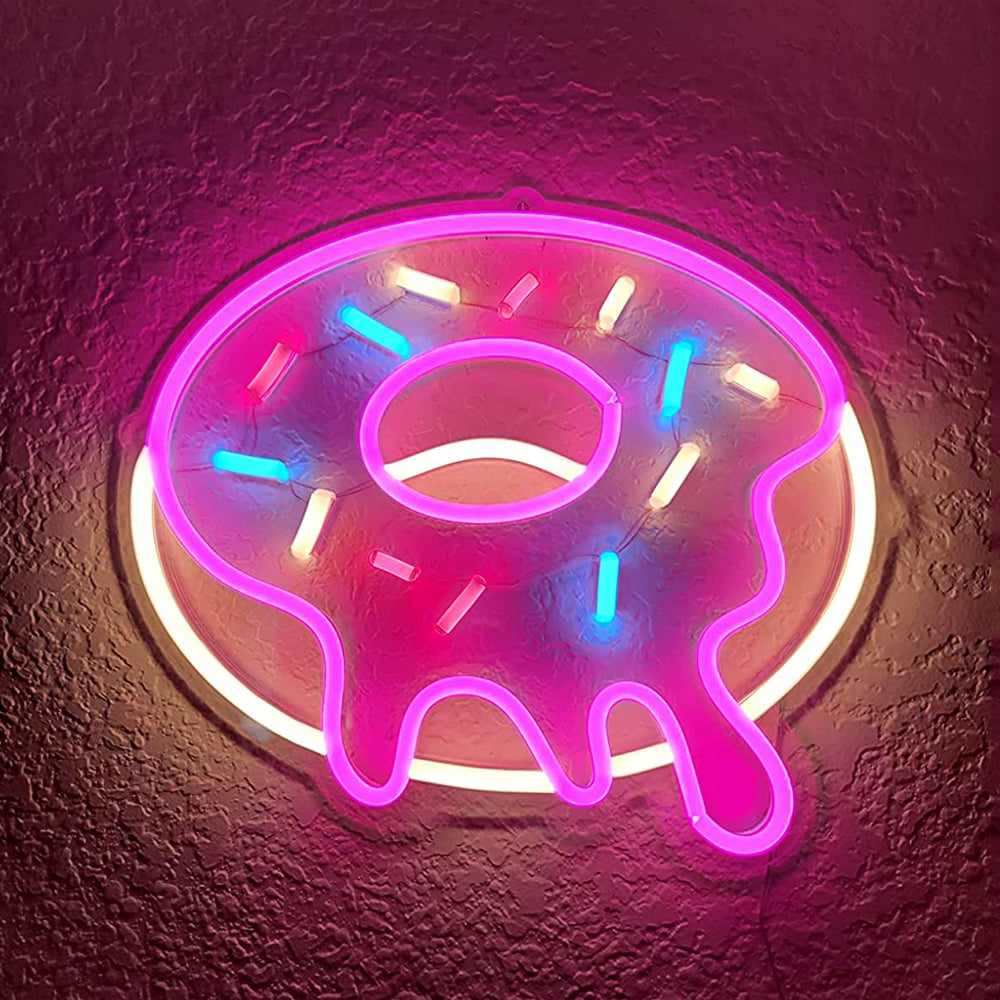A vibrant pink-frosted doughnut takes the spotlight, its glossy surface adorned with glowing sprinkles in shades of blue, yellow, and pink. The bottom part of the doughnut is a warm, golden-yellow, contrasting beautifully with the bright top. The sprinkles, reminiscent of tiny, luminous cylinders, seem to radiate warmth through their vivid colors. Behind this oval-shaped doughnut, the wall is painted a cracked pink, adding a textured backdrop that enhances the overall visual appeal.